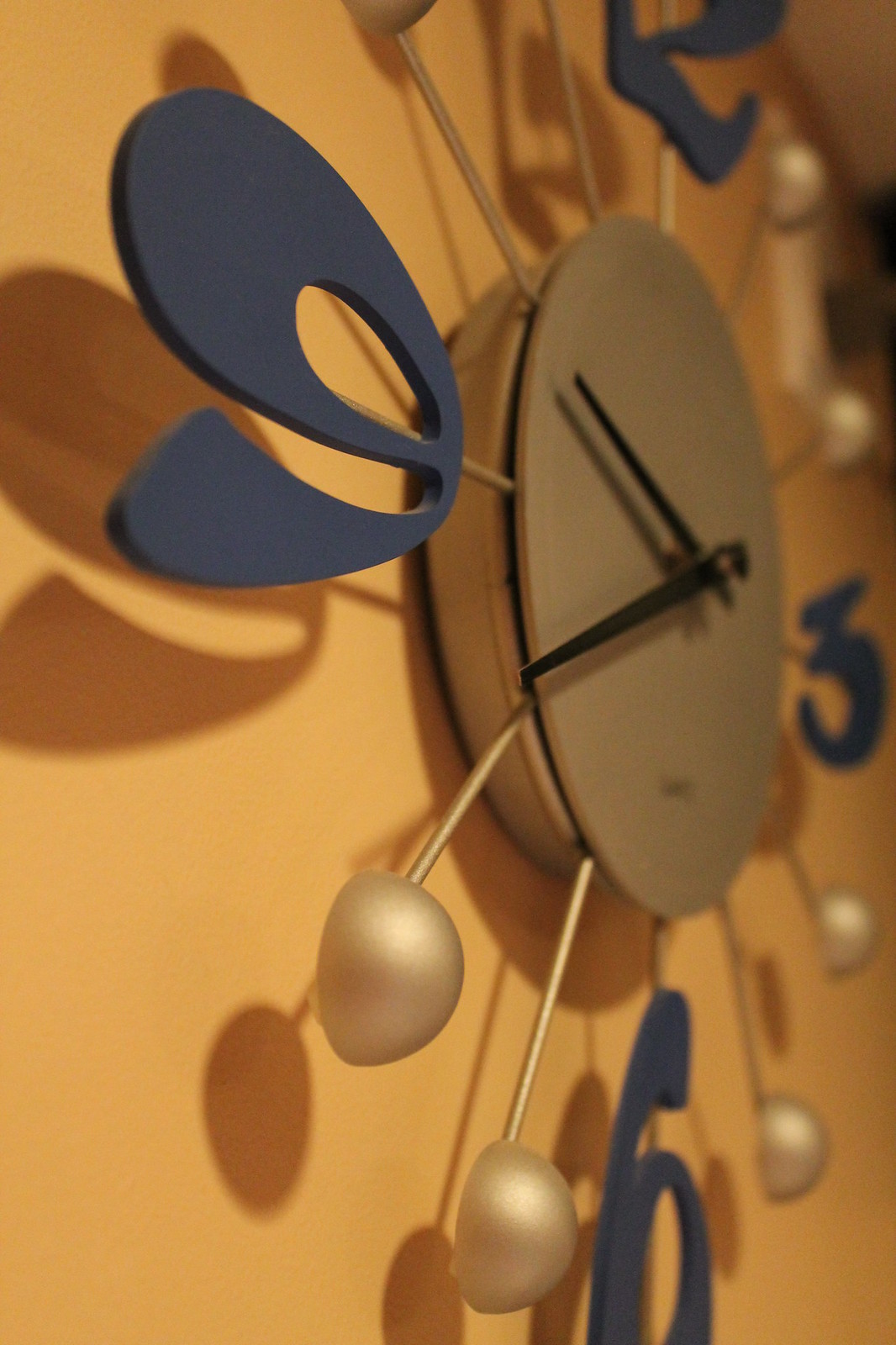The photograph captures a striking wall clock, viewed from a slight left-hand angle that highlights the prominence of the number nine. The clock features an elegant gold face without any numerical markings directly on it. Instead, the numbers are uniquely positioned on gold metal spokes extending outward. At the end of each spoke for the numbers 1, 2, 4, 5, 7, 8, 10, and 11 are small half-sphere embellishments. The numbers 3, 6, 9, and 12 are dramatically oversized, appearing inflated in design, and are colored in a deep navy blue, adding a playful contrast to the gold. The clock hands are a stark black, providing a sharp delineation against the gold face. The brand name, located at the bottom of the clock face, is unreadable in this image. All of this is set against a vibrant orange wall that enhances the clock's aesthetic appeal.